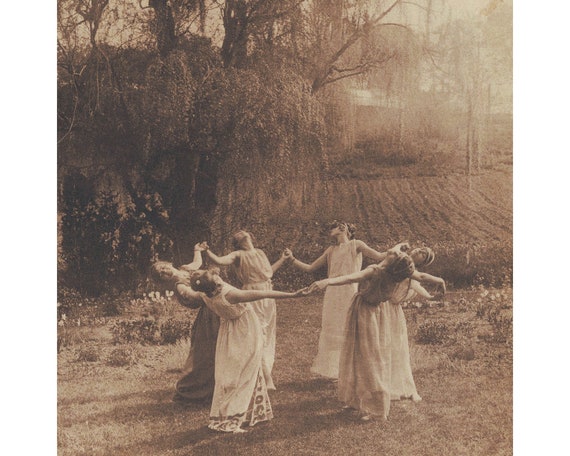This vintage sepia-toned photograph, evocative of an old postcard or book illustration, captures a group of six women wearing long white gowns or simple dresses. They stand in a circle on a bare patch of dirt, each woman's hand linked with the next, and their heads and upper bodies inclined backward as they gaze skyward. The absence of any text leaves their exact activity—perhaps performing, singing, or dancing—open to interpretation. The scene is set outdoors beneath a large willow tree with cascading leaves that nearly touch the ground. In the background, blurred by time, rows of raised vegetation—possibly grapevines—suggest a farm setting, and the hint of a house peeks through the trees. This striking image, marked by the aura of antiquity, captures a moment both serene and enigmatic.